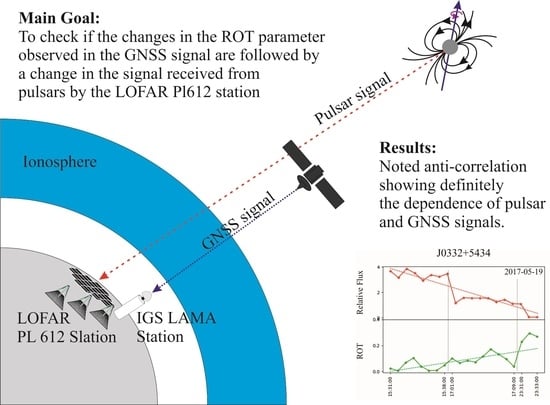The image is a detailed scientific diagram related to the study of satellite signals and their interaction with the Earth's ionosphere. In the top left corner, there is a text block specifying the main goal: to investigate whether changes in the ROT parameter observed in the GNSS signal correlate with changes in the signals received from pulsars by the LOFAR-PL612 station. The diagram features a circular illustration in the bottom left corner, with a blue-bordered outer ring labeled "ionosphere," encircling a white center marked "IGS LAMA station," and a gray inner circle labeled "LOFAR-PL612 station." Arrows point from a satellite towards the central circles, illustrating the signal pathways. Another detailed element is an apple-shaped icon indicating the PULSAR signal directed at the LOFAR-PL612 station. On the right side, the results are noted, highlighting an anti-correlation that indicates a definite dependence between PULSAR and GNSS signals. Additionally, a bar graph on the bottom right shows green lines projecting upwards and red lines downwards, visually representing the data results. This comprehensive illustration underscores the intricate relationship between various astronomical components and the corresponding GNSS signal observations.